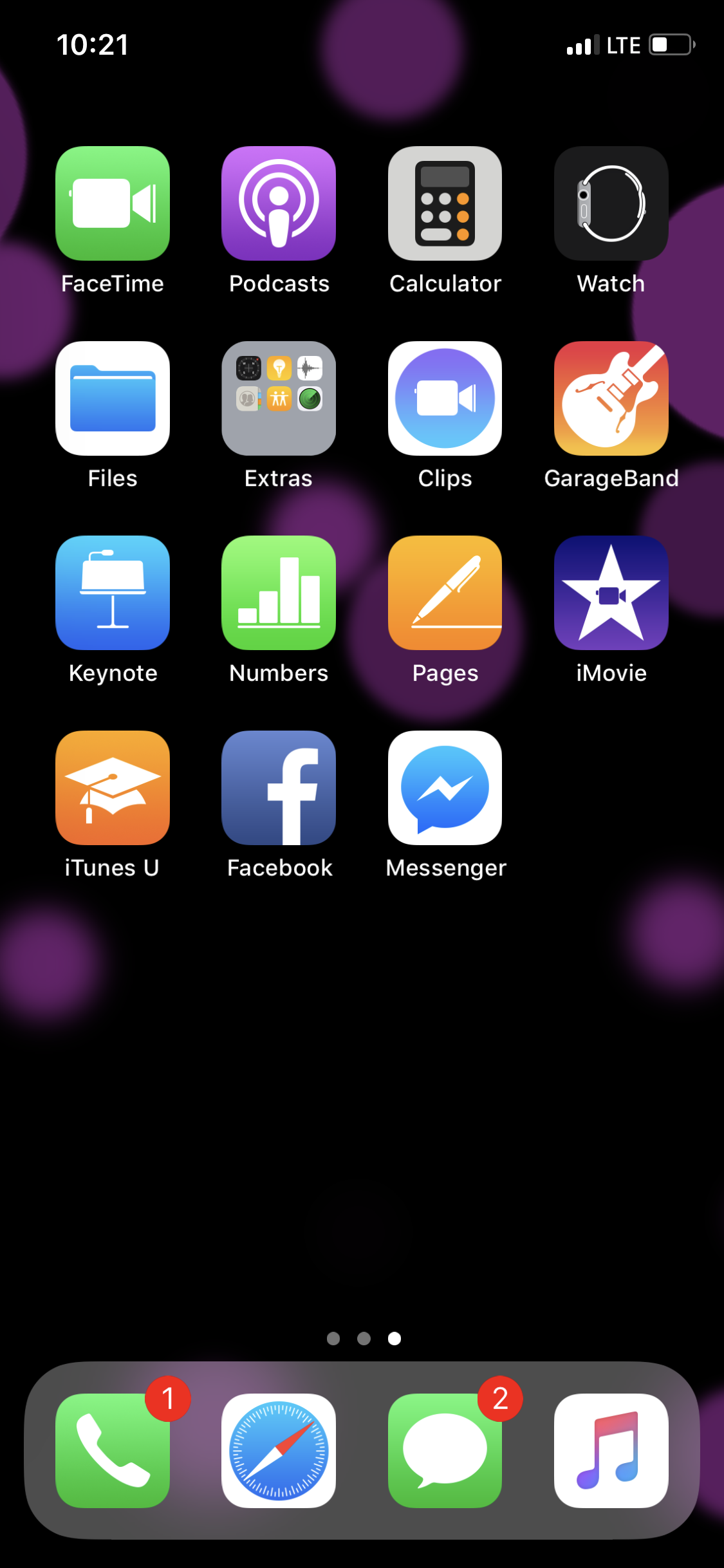This is a detailed photograph of an iPhone home screen, identifiable by its distinctive widget layout. The wallpaper features a black background adorned with numerous purple polka dots. On the top left corner, the time is displayed as 10:21, although it's unclear whether it's AM or PM. The phone shows three out of four bars of signal strength on an LTE network, and the battery indicator reveals slightly less than half a charge remaining.

The home screen itself is populated with various apps. In the first row are FaceTime, Podcasts, Calculator, and Watch. Immediately beneath these are Files and a folder labeled "Extras," which presumably contains additional apps. To the right of this folder are Clips and GarageBand. The subsequent row includes Keynote, Numbers, Pages, and iMovie, followed by iTunes U, Facebook, and Messenger in the next tier down.

At the bottom of the screen, a navigation bar displays three dots, with the third dot highlighted, indicating that this is the third and final page of the home screen.

The dock at the very bottom contains four primary apps: the Phone app (with a badge showing one missed call), the Safari web browser, the Messages app (with a badge showing two unread messages), and the Music app for Apple Music.